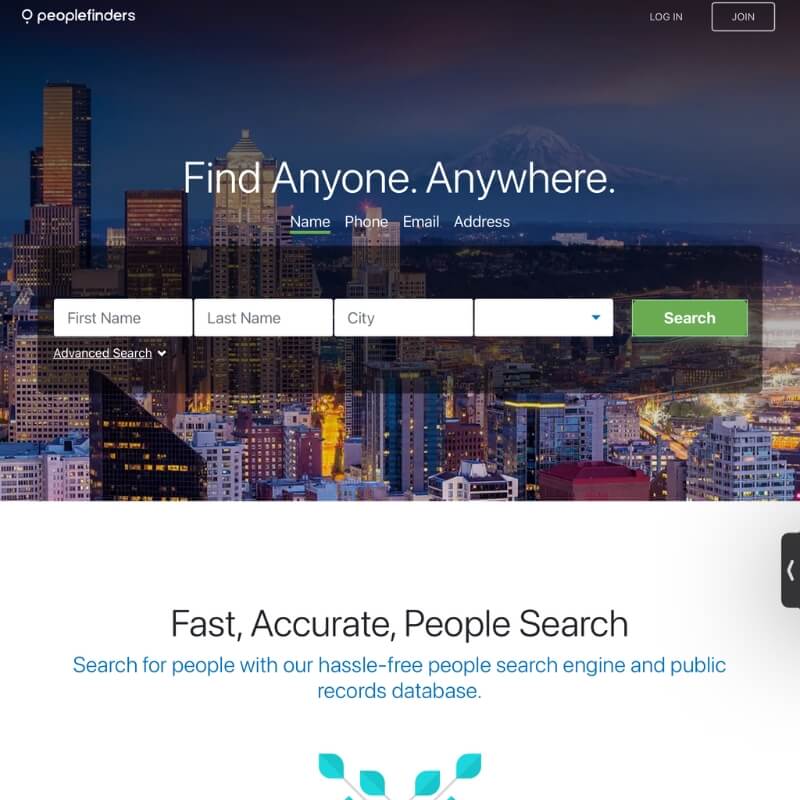The web page titled "People Finders" features a user interface designed for public searches. In the upper left corner, the title 'People Finders' is prominently displayed, while the upper right corner includes options for users to 'Log In' or 'Join'. The page has a background of a blue sky with a cityscape below, showcasing both high-rise and low-rise buildings illuminated by lights and filled with numerous windows.

Centrally located near the top of the page, above the buildings, is a bold white text stating "Find Anyone Anywhere." Below this headline, additional information prompts users to input search criteria, listing "Name, Phone, Email, Address". Beneath these instructions, there are four white input boxes labeled sequentially: "First Name", "Last Name", "City", and a blank box with a dropdown blue arrow. A prominent green search button labeled "Search" in white text is located in the center of this section.

Further down the page, right below the city scene, is a line of black text that reads "Fast, Accurate, People Search." Following this, green text encourages users to "Search for people with our hassle-free people search engine and public records database." The bottom of the page features a decorative quartet of greenish-blue leaves; two leaves face to the right and two to the left, all connected by a gray stem. This design element is centrally located and adds a touch of nature to the overall aesthetic of the web page.